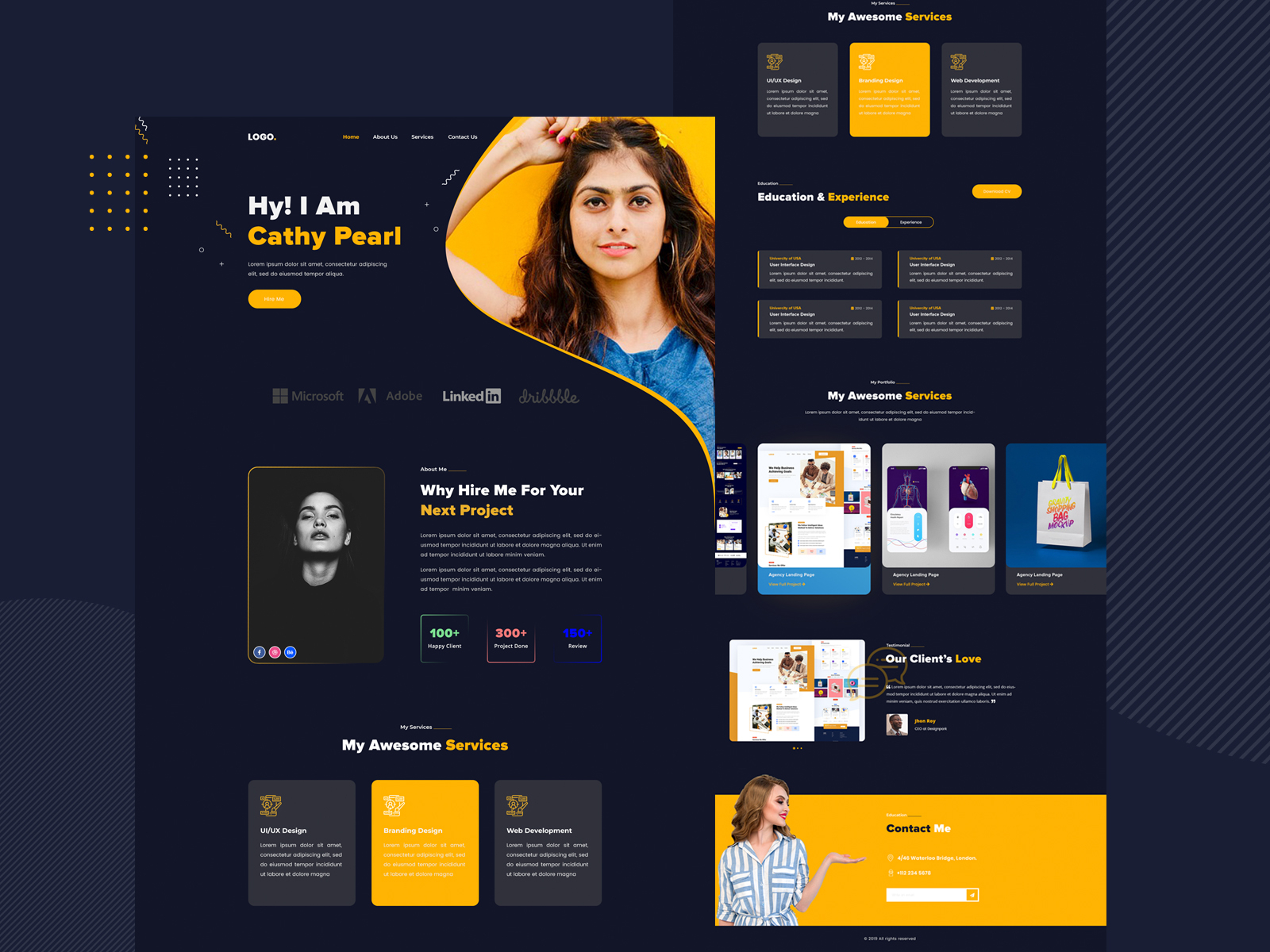This web page features a predominantly dark blue background with multiple sections displayed. On the left side, a more zoomed-in view of the main content is presented, while the right side shows a larger portion of the page, including additional vertical elements.

In the top right corner, within an orange segment, there's an image of a woman posing. The text next to her reads, “Hi, I am Kathy Pearl,” with "Kathy Pearl" highlighted in yellow. Below this is a small, difficult-to-read paragraph in white text, accompanied by a yellow button. Logos of companies such as Microsoft, Adobe, LinkedIn, and Dribbble are displayed beneath this section.

Further down the page, another image of Kathy Pearl is visible alongside a heading that says, "Why hire me for your next project?" This section includes another paragraph and a set of statistics in various colors: over 100 in green, over 300 in red, “4” with an unspecified label, and over 150 in blue.

Following this, the page lists "My Awesome Services" in three boxes with alternating colors: black, yellow, and black. Continuing on the right side of the longer page, additional sections include headings for “Education and Experience,” “My Awesome Services,” and “Our Clients Love,” each displayed within black boxes.

At the bottom of the page is an orange section with a picture of a woman pointing towards a “Contact Me” section, inviting visitors to get in touch.